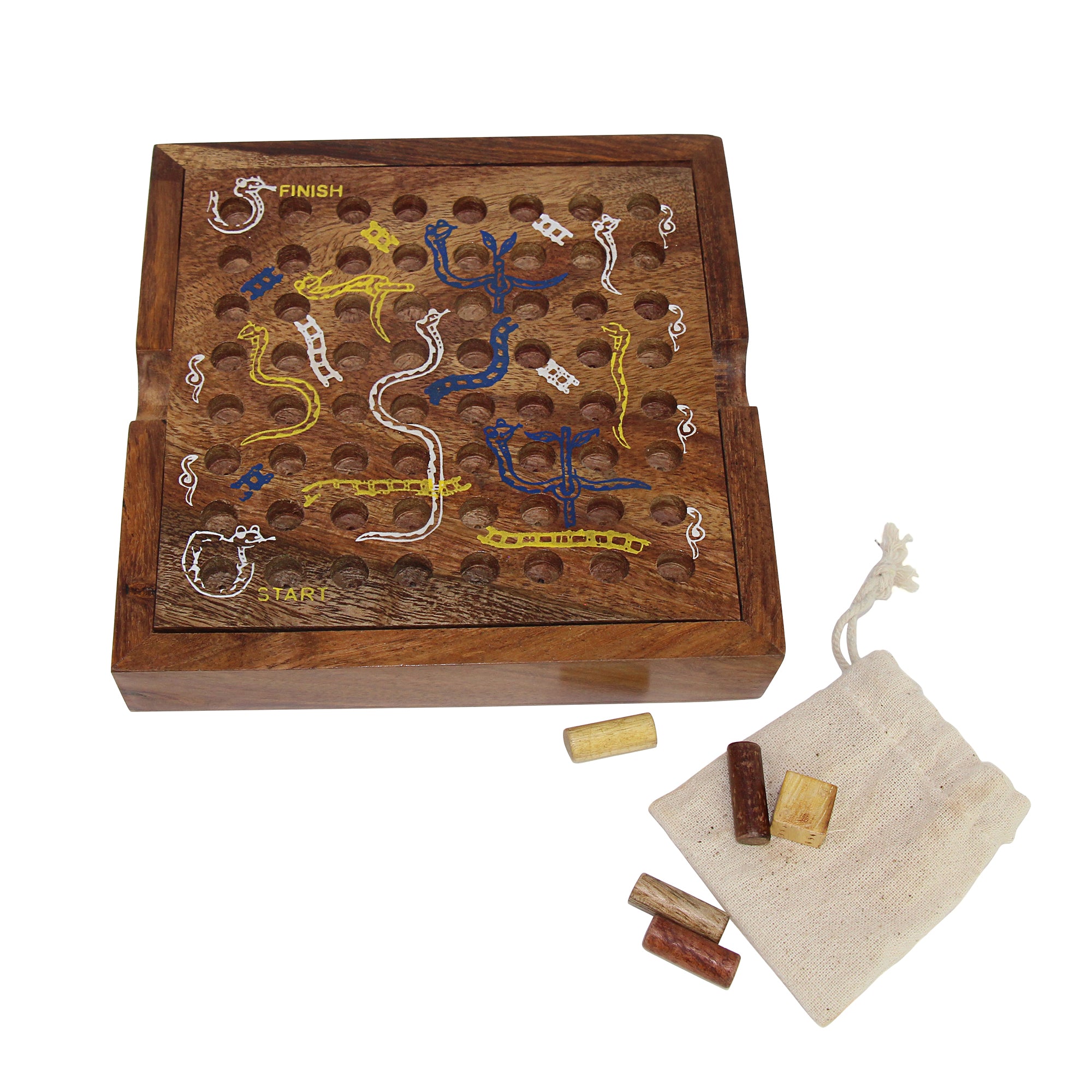This photograph captures a unique, seemingly homemade wooden game. The game board, crafted from dark brown wood, is square-shaped and features an 8x8 grid, resulting in a total of 64 holes designed to hold pegs. The pegs, varied in color, include brown, white, and tan options. On the right side of the image, a white bag is visible, presumably for storing the pegs.

The gameplay appears to be a creative variation of the classic "Chutes and Ladders" concept, using snakes and ladders instead. The board includes intricately placed white and yellow snakes, along with yellow and white bridges which players navigate during play. The game begins at the bottom left corner, marked with the word "Start" and adorned with a snake wrapping around the start peg hole. The objective is to traverse the board and reach the top left corner, labeled "Finish," which similarly features a snake surrounding the finish peg hole. This detailed, handcrafted game combines traditional elements with a novel design, making for an intriguing and visually appealing piece.